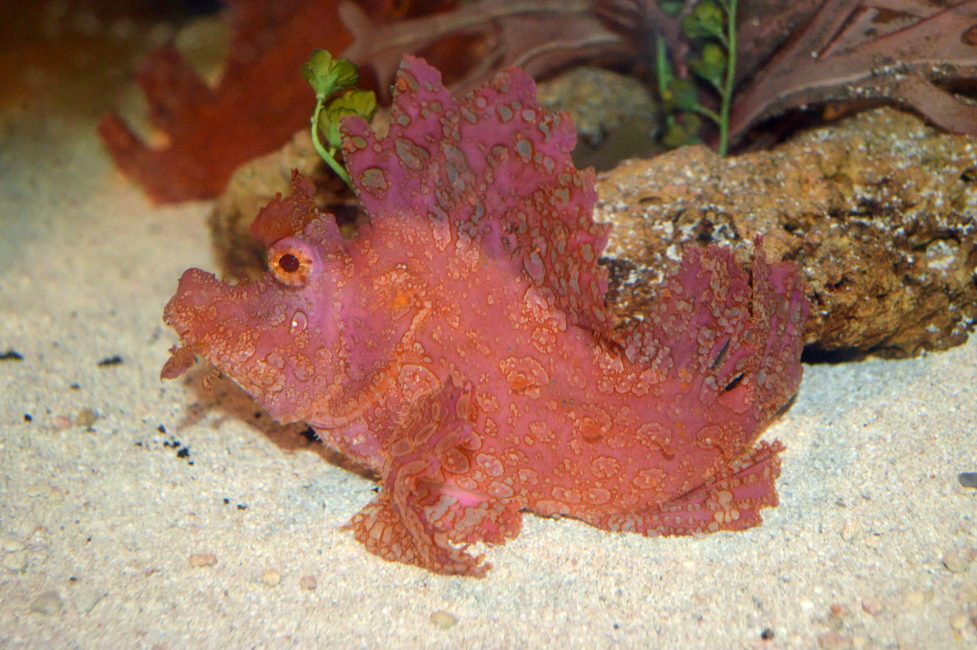This photograph captures a striking and unusual fish resting on the sandy bottom of what appears to be an aquarium. The fish is predominantly red with varying shades of purple and orange, making it stand out vividly against the beige, pebble-like sand. Its body exhibits unique, abstract patterns that resemble coral, with jagged fins that give it a frilly, almost plant-like appearance, akin to cabbage leaves. The fish's large, golden-orange eyes with black pupils add to its distinctive look. The fins, which are somewhat transparent, fan out in a way that helps the fish navigate the seabed. You can see only one side of the fish, emphasizing its sideways position. Behind the fish are blurry elements, including rocks and a sprig of a plant, reinforcing the idea that this is indeed an aquarium setting. The fish's appearance suggests it would be well-camouflaged in a coral reef environment due to its coral-like features.